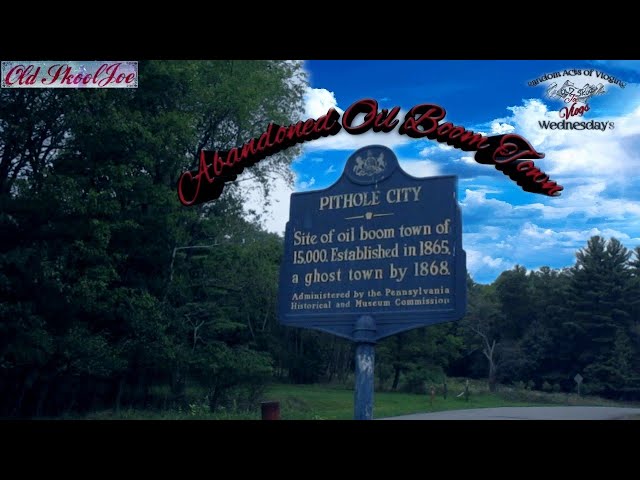The image depicts a sign at the entrance of Pithole City, a historical ghost town and former oil boomtown that once had a population of 15,000, established in 1865 and abandoned by 1868. This sign, made of dark metal with yellow or gold inlay, is administered by the Pennsylvania Historical and Museum Commission, indicating its current status as a historical site. The setting shows a rural, picturesque landscape with an abundance of greenery including tall conifers, leafy trees, and a maple tree, all appearing under a bright blue sky with white clouds. In the background, there's a road running to the right, framed by lush grass and trees, enhancing the sense of a serene, preserved historical location. Some additional text, such as "Old School Joe" in red and "Wednesdays" can be seen, suggesting that this image might be part of a program or video frame, potentially used in media or tourism promotion.